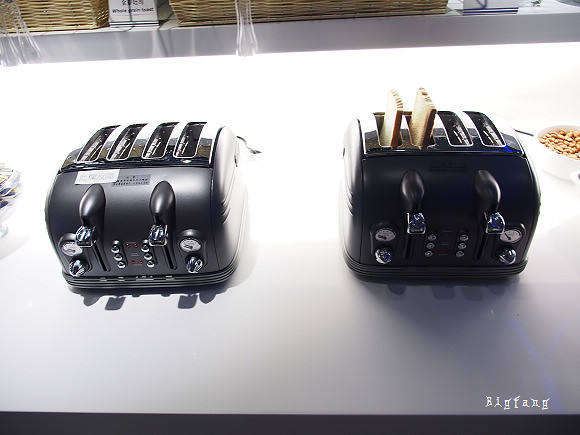This photograph captures a top-down view of two identical, high-tech black toasters placed side-by-side on a bright white countertop that appears to be part of a commercial kitchen or breakfast bar setup. Both toasters have four slots each, with the one on the right featuring two pieces of bread sticking out, though it is unclear if they are toasted or awaiting toasting. The toasters each come equipped with two levers and various settings and buttons. Above the toasters, shelves are visible holding baskets, which likely contain breakfast items or plates. To the right of the rightmost toaster, there's a white bowl, possibly filled with cereal, though its contents are somewhat obscured. The countertop is illuminated by lights under the shelving, making the surface appear very bright. At the bottom right corner of the image, the name "Big Thing" or "Big Fang" is credited, distinguishing the image with a brand or creator's mark.